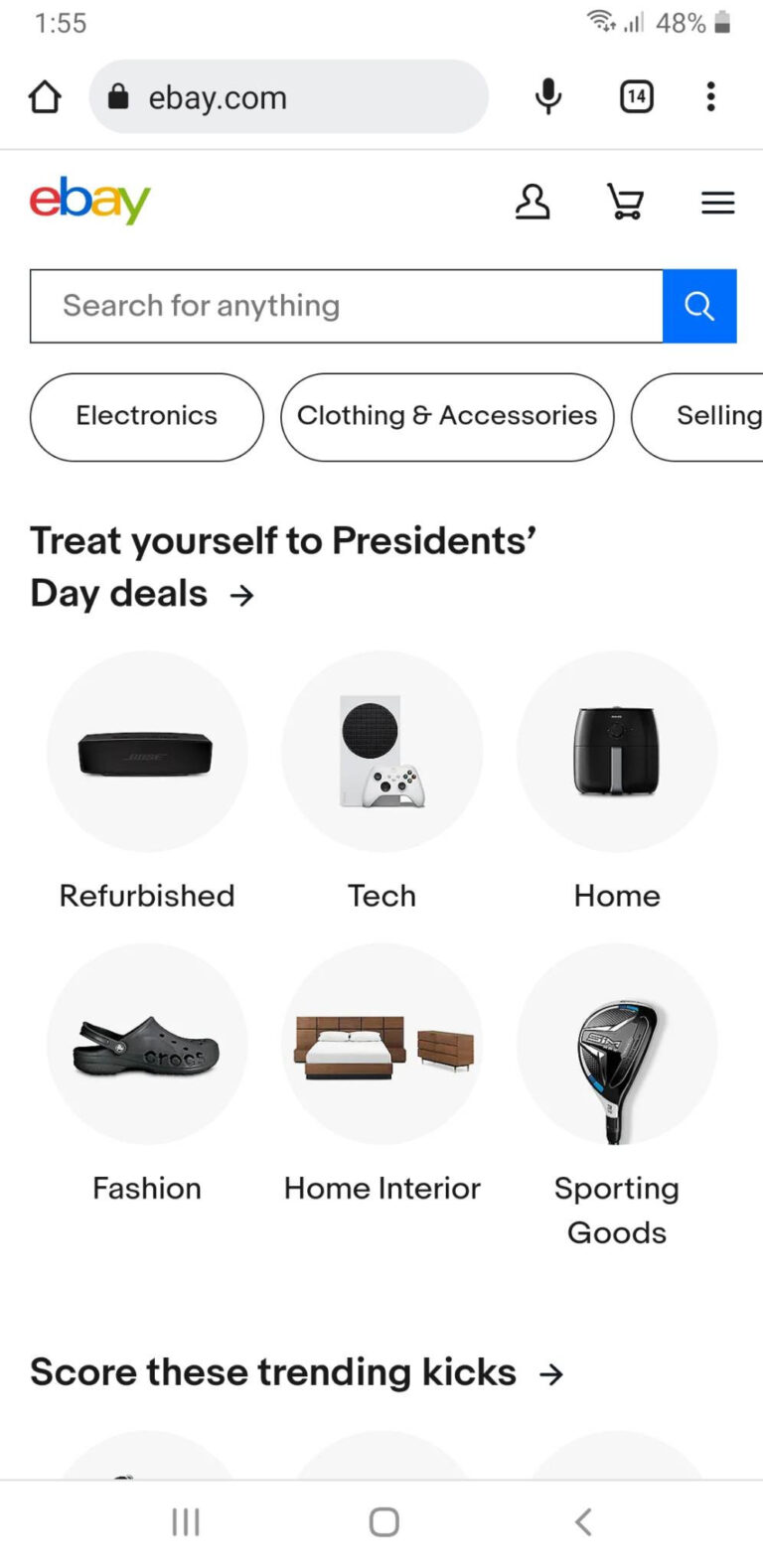A vertically rectangular screenshot of a smartphone screen displaying eBay's homepage. The top of the screen features a white background with user interface elements: the time "1:55" is displayed in the top left corner, and the top right corner includes icons showing Wi-Fi signal strength, "48%" battery life, and a battery icon. Below this, the URL "ebay.com" is visible alongside a microphone icon and an indicator showing "14" open windows.

Centered under the URL, the recognizable eBay logo is positioned on the left, with icons for the user profile, shopping basket, and menu arrayed to the right. Directly below, a search field invites user input. Further down, three horizontal buttons labeled "Electronics," "Clothing & Accessories," and "Selling" offer quick navigation options.

The main promotional banner reads "Treat Yourself to President's Day Deals," immediately followed by two rows of circular images. These images, categorized under headings such as "Refurbished," "Tech," "Home," "Fashion," "Home Interior," and "Sporting Goods," highlight various product categories. Finally, at the bottom of the screen, a section titled "Trending Kicks" is marked with an arrow pointing right, indicating more content available.